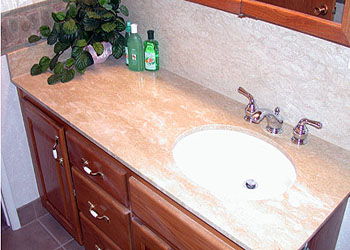This image showcases a meticulously maintained vanity with a sophisticated beige and brown color scheme. The countertop, made of granite, is incredibly smooth and polished, reflecting light and adding an element of elegance to the setting. The vanity itself is constructed from brown oak, featuring a refined, glossy finish that enhances its natural beauty. The cabinet handles are a rich rust color with white, decorative beaded accents in the center, contributing to the overall aesthetic appeal. 

To the right of the vanity, part of a large mirror with a matching dark wood trim is visible, adding continuity to the design. In the corner of the countertop, a lush green plant brings a touch of nature into the space. Adjacent to the plant, a tidy arrangement of personal hygiene items, including shampoo, conditioner, and mouthwash, are neatly placed. The sink, centrally located, boasts sleek silver handles and a pristine white basin, further emphasizing the cleanliness and orderliness of the area.